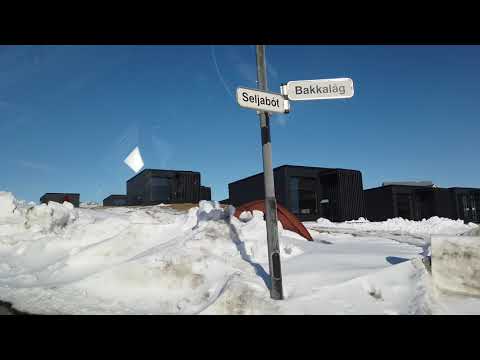The image portrays a snowy, outdoor scene in the middle of the day, characterized by a thick snow blanket approximately 15 inches deep covering the ground. Dominating the center of the image is a metal street sign pole with two signs; the left sign reads "Sai Jabot" and the right sign reads "Baka Log." The background features a series of black metal shipping containers, some of which appear to have windows. The contrast between the snowy foreground and the clear blue sky devoid of clouds highlights the coldness of the setting. Overall, the image, being grainy and blurry, emphasizes the starkness and repetition of the black containers against the pristine white snow, creating an almost monochromatic scene with sporadic splashes of blue, brown, and gray.